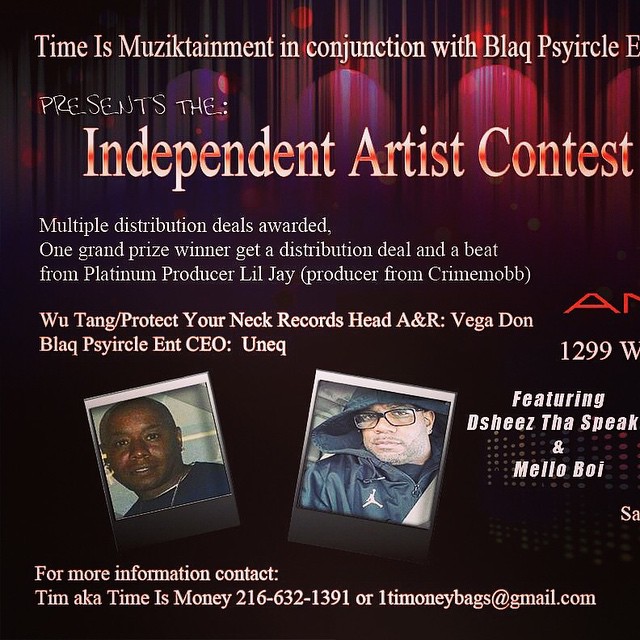The image is a partially cut-off flyer promoting an "Independent Artist Contest." The background features red stage curtains with circular stage lights in black, purple, red, and blue hues. At the top, it states "Time is Muztainment in conjunction with Black Spherical Entertainment presents the Independent Artist Contest." The main highlight reads, "Multiple Distribution Deals Awarded," with a grand prize of a distribution deal and a beat from platinum producer Lil' Jay, known from Crime Mob and Wu-Tang's Protect Your Neck Records. 

Additional details include Vega Dawn as Head A&R of Protect Your Neck Records and Black Spherical Entertainment's CEO UNEQ. There are two Polaroid-style pictures at the bottom: one shows a man in a dark blue shirt, and the other depicts a man wearing a Jordan jacket with a hood, glasses, and facial hair. The names "Featuring DeShea's The Speak and Mellow Boy" are linked to these images. For more information, contact Tim, aka Time is Money, via phone number 216-632-1391 or at timoneybags@gmail.com.